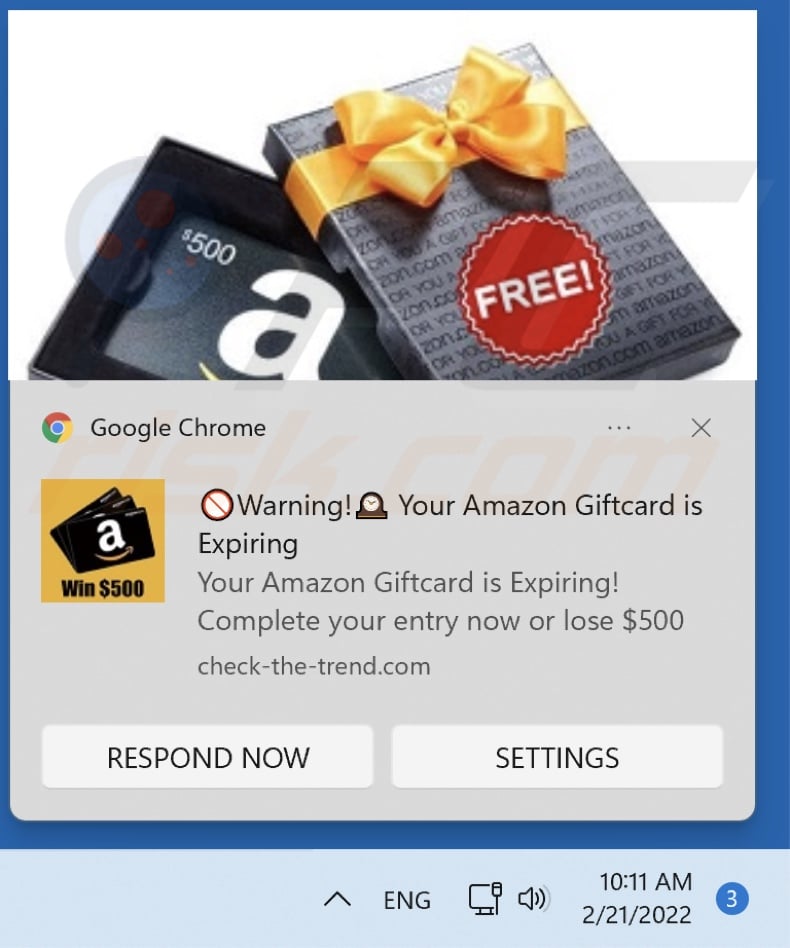This image features a dark blue border framing a promotional graphic. At the top, there is a photograph of an open gift box containing an Amazon gift card valued at $500. The gift box lid, which is gray with a shiny yellow bow, is placed on top of the bottom part of the box. A red decal labeled "FREE" in white letters, with "Google Chrome" written underneath, is also visible on the lid. Below this is a dark yellow square showcasing three illustrated Amazon gift cards, and adjacent text that reads "Win $500."

A prominent warning is displayed below, featuring a circle with a red slash and the word "Warning!" accompanied by an emoji of a clock. The message warns, "Your Amazon gift card is expiring. Complete your entry now or lose $500," redirecting viewers to "Check-the-trend.com." Instructions to "Respond now" are visible alongside "Settings."

In the bottom right corner, the display shows "ENG," a volume button, and a timestamp reading "10:11 a.m. 2-21-2022." Additionally, a blue circle with a white number "3" is centered within it. The image does not contain any people, animals, plants, flowers, or trees.